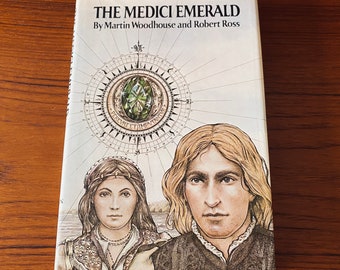The image is a detailed cover of the book "The Medici Emerald" by Martin Woodhouse and Robert Ross, resting on a wooden desk with an ambery brown or middle brown oak finish. The book's title is prominently displayed at the top in black text. The cover features an illustration of two white-skinned, Caucasian individuals—a man with long, golden blonde hair and a slight 5 o'clock shadow, wearing a tunic, and a woman with lighter brown hair and a headband, adorned with several rows of pearls. Both characters share similar facial features, with the woman also depicted in a collared outfit. Central to the cover design is an elaborate compass with a jewel in the center, adding a touch of mystery and adventure to the aesthetic. The background of the cover is white, contrasting sharply with the detailed drawing and text.